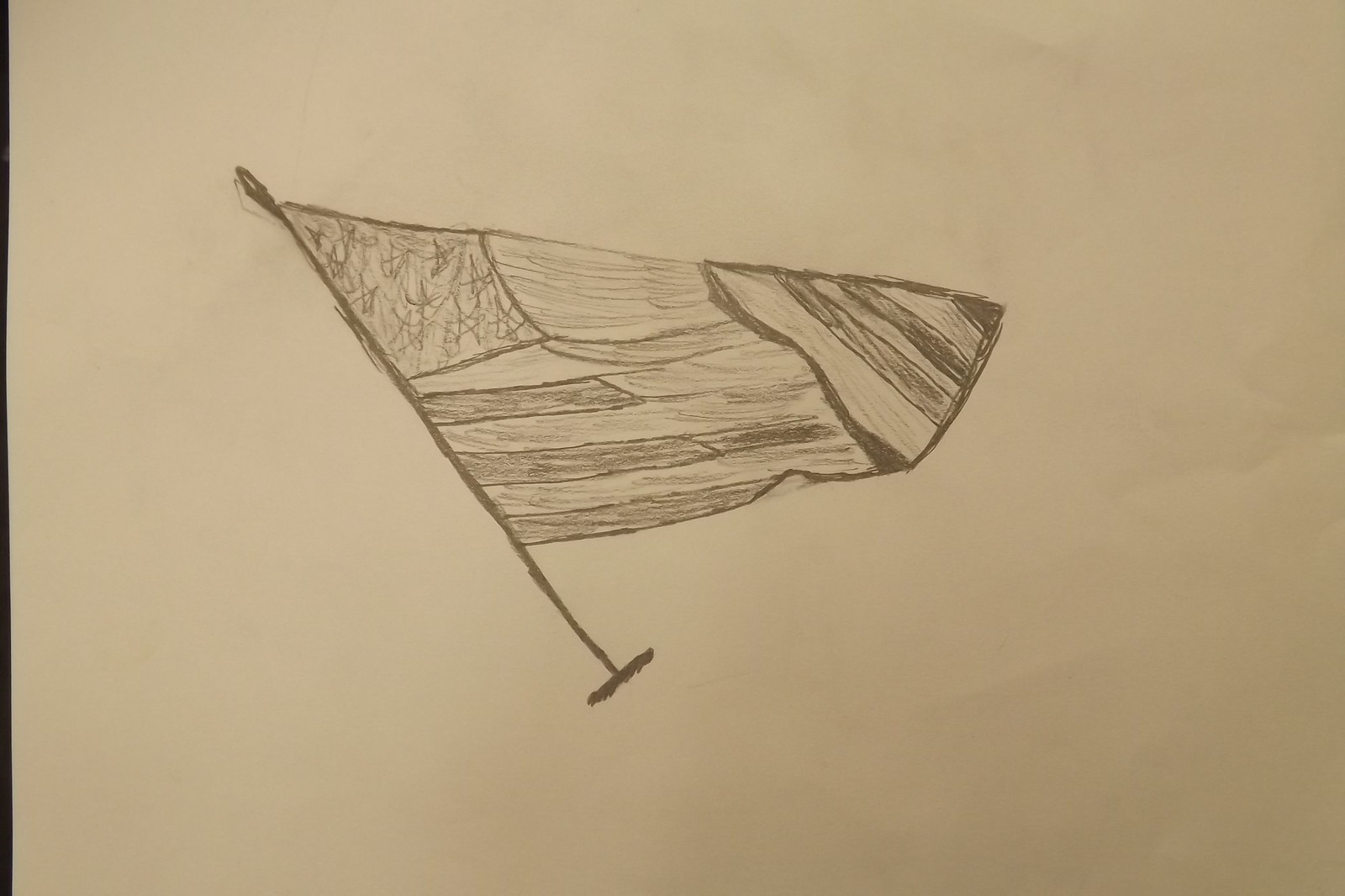An intricately detailed pencil drawing is centered on an off-white background, depicting a potential flag design. The flagpole is represented by a prominent black line, suggesting the flag is fluttering outward in the wind. The flag features a pattern of pencil-sketched stripes, with three horizontal stripes crossing its width and two vertical stripes spanning its height. At the upper left corner, a small square filled with penciled stars is meticulously shaded, adding a touch of complexity to the sketch. The entire drawing is executed in light black pencil, showcasing fine shading that gives depth and dimension to the design.